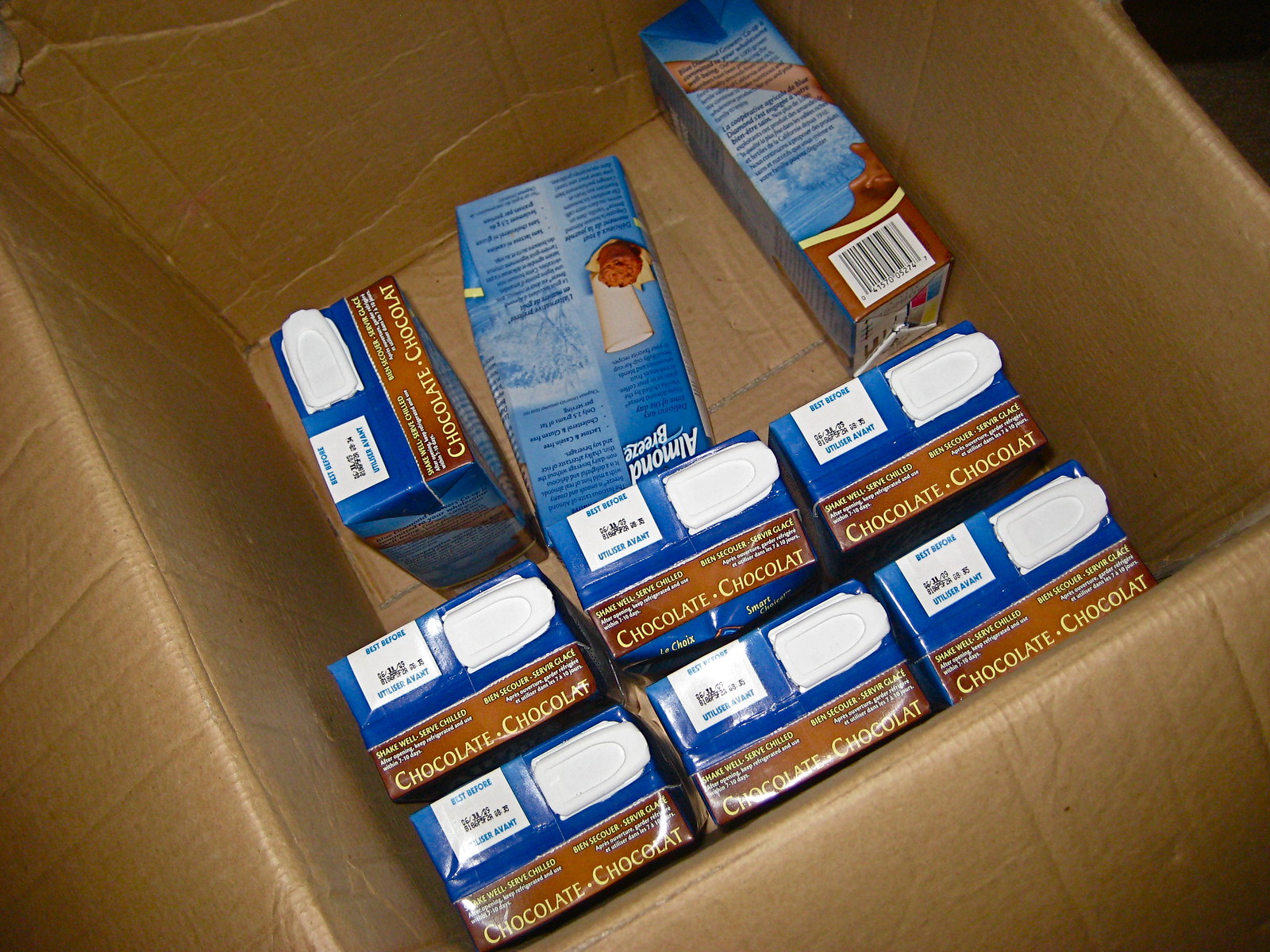The image depicts the inside of a large, brown, cardboard box that is open, showing its contents from an aerial point of view. The box seems oversized relative to its contents. Inside, there are nine identical packages of what appears to be shelf-stable almond milk labeled as "Chocolate Chocolat." Six of these packages are neatly lined up at the bottom of the box, all displaying a bright blue shiny label with a brown band and gold writing. Each package prominently features the word "Chocolate" in English and "Chocolat" in French, and includes white sticker labels on its left side along with visible expiration dates and spouts.

Above these six packages, three additional identical packages are positioned differently. One stands vertically but is angled 90 degrees from the others, another lies flat on its front face revealing the back of the box with an upside-down label, and the third rests on its side, tilted against the side of the box. In the upper right corner of the large box, there is an open area showing the bottom of the box, emphasizing the sparse and somewhat disordered arrangement of the items inside.